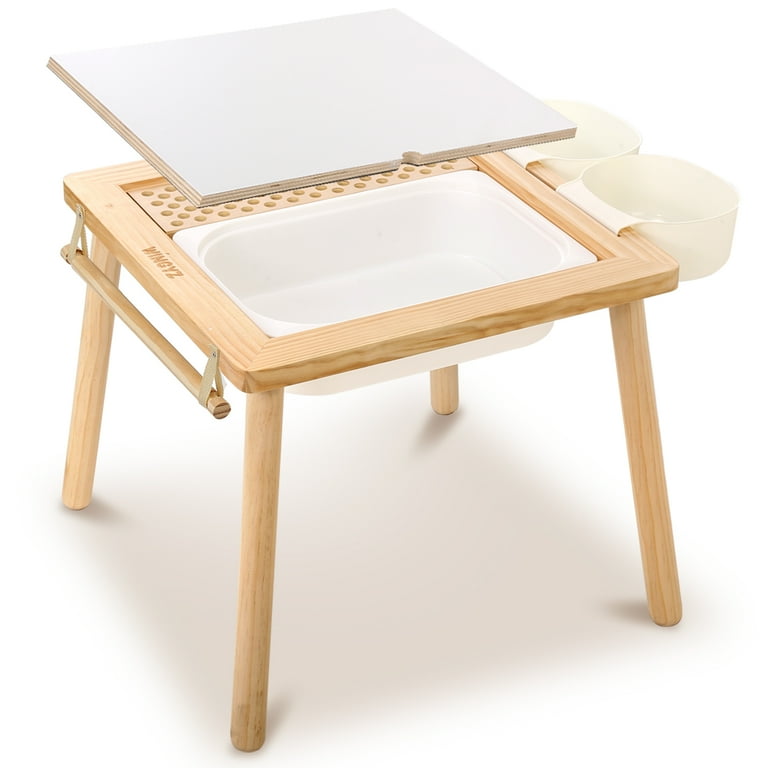The image showcases a multifunctional small wooden table, appearing almost like a footstool, crafted from very light tan, unfinished wood with rounded legs. The table features a variety of practical attachments and compartments. On the left side, a wooden dowel is suspended from the side by two leather straps, suitable for hanging a towel. The right side is equipped with two small beige plastic cups attached via slits, possibly for storing small items. The top of the table holds a white plastic bin, partly concealed by a removable wooden piece with punched holes, potentially serving as a cutting board or for food storage. Additionally, the upper surface incorporates a contrasting section, a flat piece that could be ceramic or another type of material, providing an additional utility feature. The overall design is clean and simple, possibly indicating the table’s use in a cleaning station or a multifunctional household item setup.